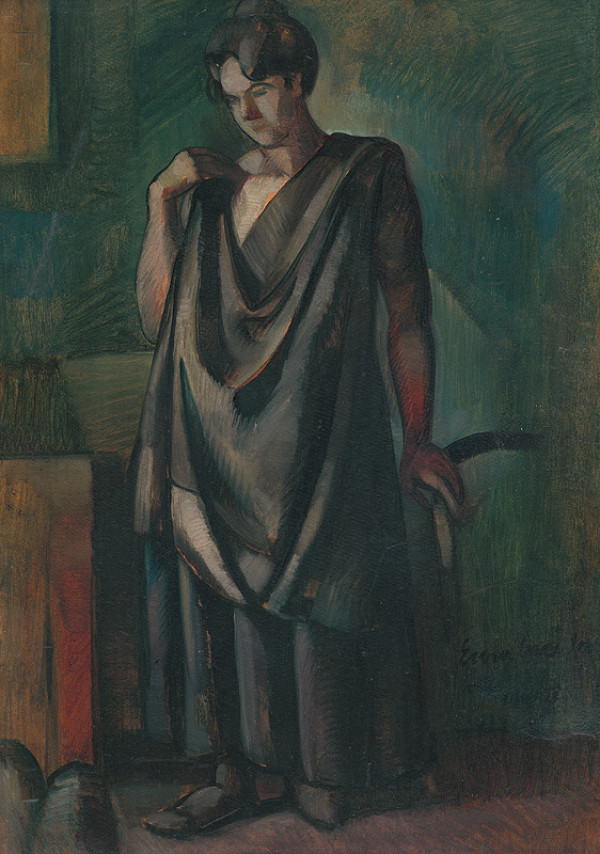The image portrays an art piece featuring a woman with short black hair, rendered in intricate colored charcoal. She is attired in a dark dress resembling traditional Southeast Asian or South Asian clothing, which flows into a skirt. Her complexion is white, and her pose includes resting one hand on a green chair with black wooden borders, while her other hand touches her shoulder. The background is a textured green wall, possibly greenish blue, which also includes some abstract shapes towards the bottom left and a window at the top left. Beside her, on the left side of the image, there is a table. Her gaze is directed downwards, adding to the contemplative atmosphere of the piece. Though the artist’s signature appears above the bottom part of the painting, it remains unclear.